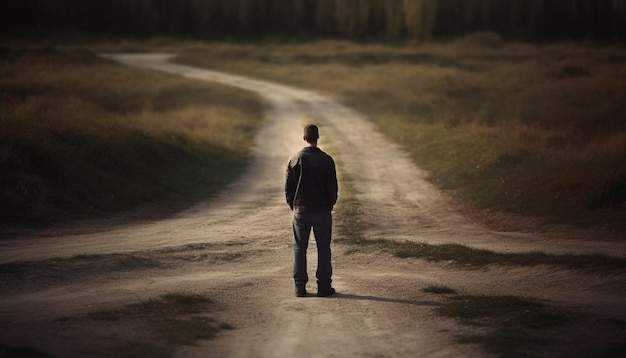In a dusky, autumnal landscape, a lone man stands at a crossroads of dirt roads, captured from behind. Cloaked in a dark gray jacket and matching pants, with his hands possibly in pockets, he seems to be contemplating the path ahead. The scene is shrouded in dim light, making it hard to discern his exact features, though his short, dark hair is faintly visible. To his right, his shadow stretches across one of the dirt roads. The crossroads comprise a primary path extending before him that gently curves left and ascends, flanked by side roads branching off to the left and right. The entire area is enveloped in thick, lush green grass and tall vegetation, contributing to an overarching sense of solitude and desolation. In the distance, a dark, almost opaque bar spans the horizon, enhancing the overall impression of isolation. The photograph powerfully encapsulates the man's solitary moment, underscored by the barren, unpaved roads and the encroaching wild foliage.